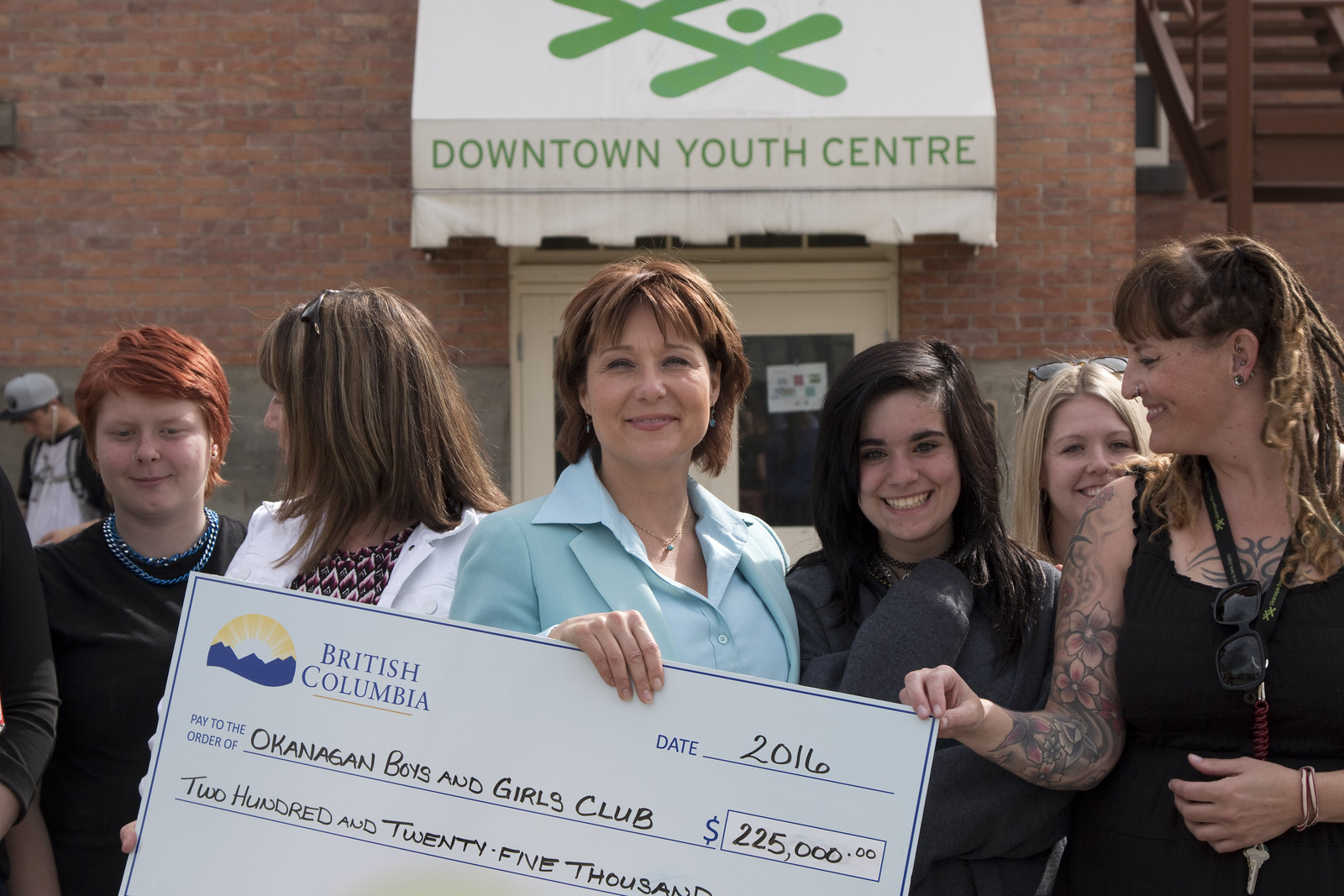In this daytime outdoor photograph, a group stands in front of a brick building with a white eaves that reads "Downtown Youth Center" in green print. Central to the image, a light-skinned woman with short, straight, choppy brown hair, adorned with light pink lipstick, smiles directly at the camera. She wears a light blue dress jacket over a button-up collared shirt, revealing a necklace. She holds a large check prominently displayed in front of her, with text that reads "British Columbia," dated 2016, paid to the order of "Okanagan Boys and Girls Club," in the amount of $225,000. 

Flanking the central woman, on the left, a young girl with flaming dyed red hair wearing a black shirt and blue chains around her neck stands next to another woman. The second woman has her head turned away, displaying scraggly brown hair. To the right, a young teenage girl with dark brown hair also smiles at the camera. Behind her stands a girl with light blonde hair and Caucasian skin. On the far right, a woman possibly in her 30s or 40s, sporting tattoos and dreadlocks, looks towards the central woman while helping to hold the check’s corner. The group’s attire is mostly black, contrasting with the central woman's light blue outfit, with their skin tones and the colorful elements, such as the red hair and blue chains, adding vibrancy to the scene.